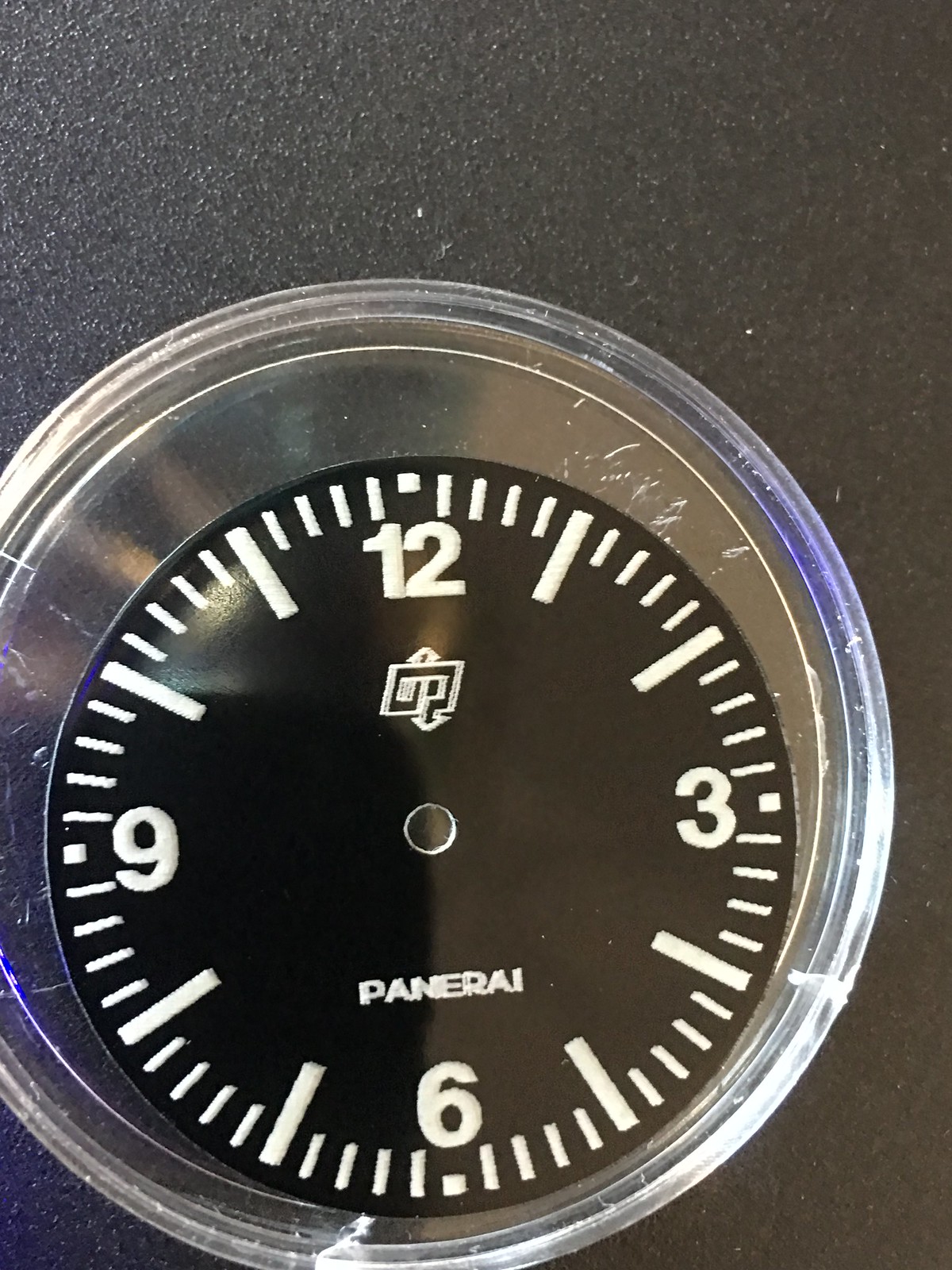Caption: "The image showcases a cut-off view of a sophisticated Panerai clock dial against a deep black background. The clock features an elegant silver bezel and a circular glass front. The black face of the clock is marked with crisp white numerals for the hours 12 through 11 and corresponding seconds. Notably, the clock lacks hour, minute, and second hands, resulting in no indicated time. The brand name 'Panerai' is prominently displayed in sleek white lettering at the 6 o'clock position, adding a touch of luxury to the timepiece."